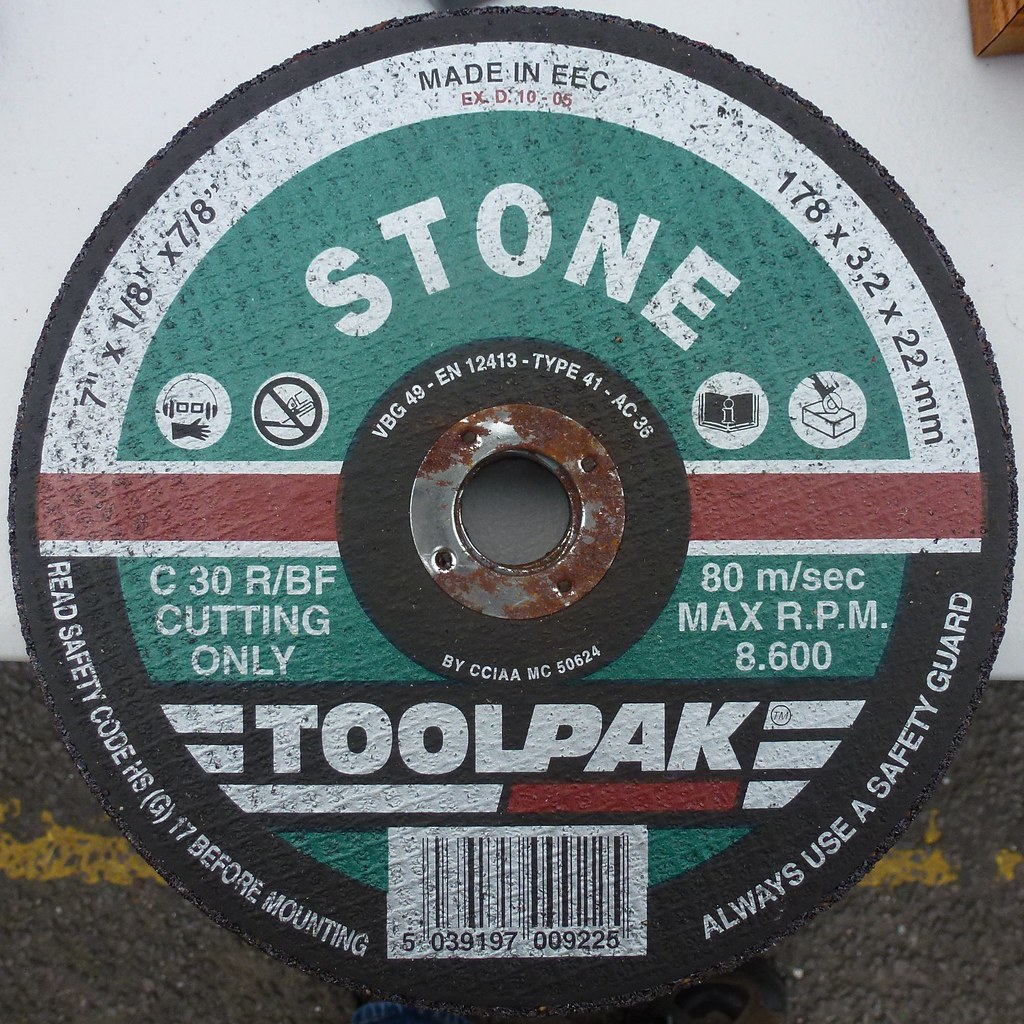The image showcases a square frame with a saw blade prominently featured against a grainy, rock-like gray-brown background, adorned with a horizontal yellow stripe resembling a roadway. The saw blade itself is circular with a black outline and an inner green circle. A red horizontal stripe runs through the green section, which bears the word "STONE" in bold white print. Below this, the words "TOOLPACK" are visible, alongside various technical descriptions.

At the top of the saw blade, set against a white background, it reads "Made in EEC" in black print. Adjacent are additional specifications: "7 inches by 1/8 inch by 7/8 inch (178 x 3.2 x 22 mm)." Below this, in red print, the code "6XD10-05" is noted. There are also four small white circles containing safety icons. Alongside the barcode at the bottom, cautionary instructions read: "Read safety code HSG 17 before mounting. Always use a safety guard."

Further text across the blade includes: "C 30 R/BF cutting only, 80 M/sec, max RPM 8600", and a metal partition stating "BBG4NEN12413 type 41AC36 by CCIAA MC50624." The detailed barcode "5039197009225" completes the informative annotations on the saw blade.